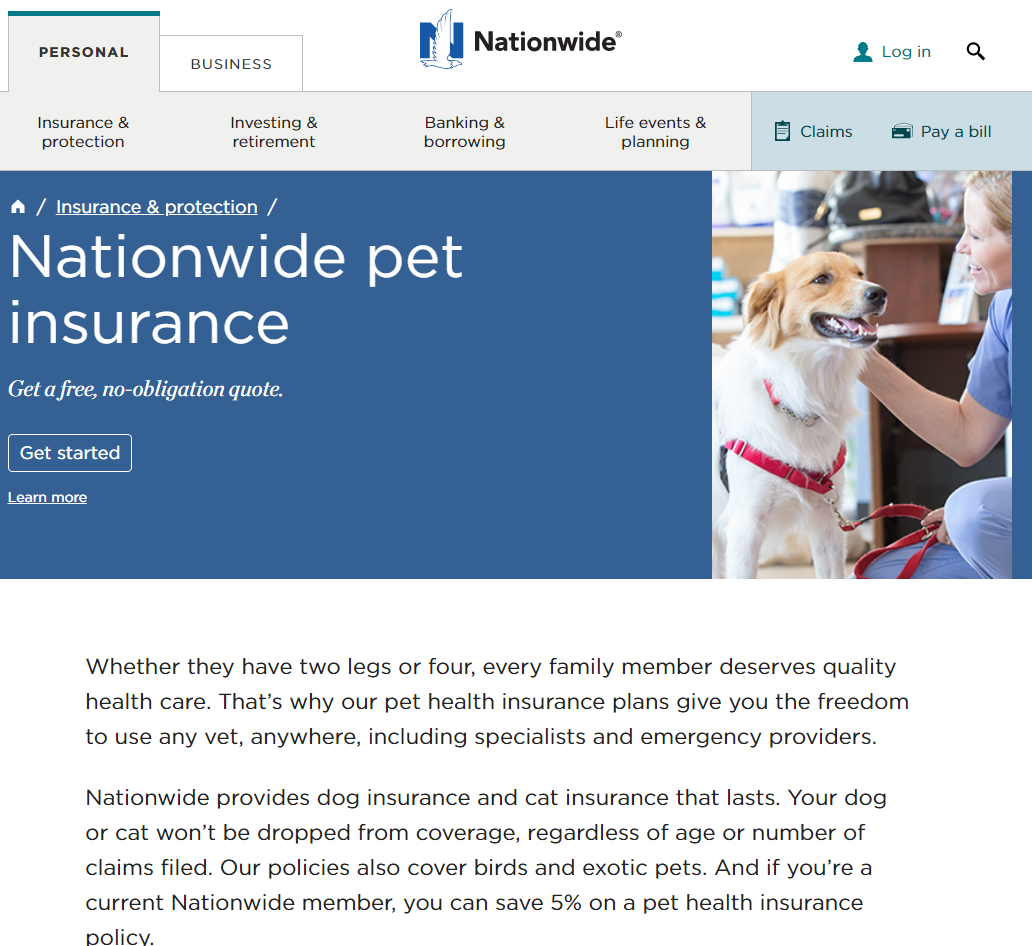This image is from the Nationwide website, showcasing a webpage layout. The top portion of the page is white, followed by a gray bar underneath it, and the rest of the page is a vibrant blue. Across the top, there are tabs labeled 'Personal' and 'Business.' Centrally located at the top is the Nationwide logo, while the top right corner features 'Login' and 'Search' buttons.

Under the 'Personal' tab, several categories are listed: 'Insurance and Protection,' 'Investing and Retirement,' 'Banking and Borrowing,' 'Life Events and Planning,' 'Claims,' and 'Pay a Bill.' 

In the navy blue section of the page, on the left side, it highlights 'Insurance and Protection,' with a specific mention of 'Nationwide Pet Insurance.' There's an invitation to 'Get a free no-obligation quote,' along with 'Get Started' and 'Learn More' buttons.

On the right side of this section, there is an image of a veterinarian technician petting a brown and white dog, which is equipped with a red leash and harness. At the very bottom of the image, black text discusses the importance and quality of pet insurance.